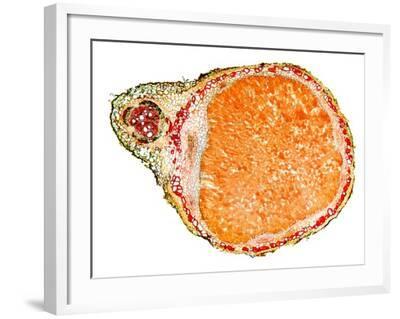This image is a detailed color photograph of a scientific illustration or microscopic organism, set within a simple white frame. The frame is tilted slightly to the right and features a white background with small shadows and gray lines on the edges. Within this frame is a cross-section of what appears to be an organic object or a magnified cell. The main portion of the object is a large, irregular orange mass with a darker orange on top and lighter towards the bottom. It is bordered by multiple rings: an inner white ring, a middle ring of red dots forming a dotted line, and a lighter gray line on the outer edges. To the left of the orange mass, a greenish appendage protrudes, containing a red circular center. The object’s overall shape is somewhat amoeba-like, almost resembling a sideways pear with a bulbous extension on its left side. This highly detailed and colorful illustration lacks any labels or text, suggesting it might be a stylized or artistic representation of cellular structures or biological tissue.